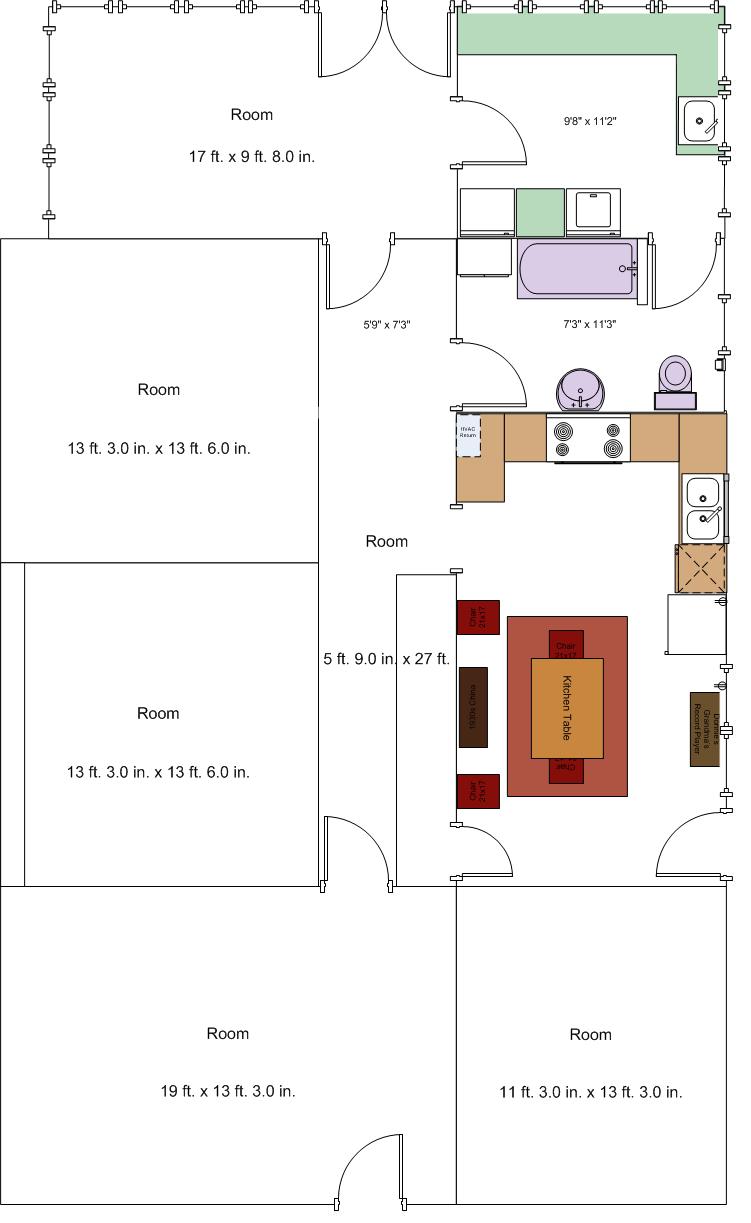The image depicts a floor plan of a house, roughly rectangular in overall shape. 

At the very top left corner, a small room is labeled "Room," measuring 7 feet by 9 feet, accompanied by an unreadable note marked "8.0." To its immediate right is another square room with green highlights along the upper and right sides and contains some small, unreadable measurements.

On the left side of the floor plan, positioned vertically, are two identical square rooms stacked atop one another. Both rooms are labeled "Room" and measure 13 feet, 3.0 inches by 13 feet, 6.0 inches.

Directly below these rooms extends a larger rectangular room with a distinctive curved cutout in the lower right corner. This room is labeled "Room" and measures 19 feet by 13 feet, 3.0 inches.

Adjacent to this, on the right side, is another small rectangular room with a few purple shapes. This room appears to feature a bathroom setup, including a bathtub at the top, a sink below it, and a toilet in the bottom right corner. Like the others, it has unreadable measurements.

Beneath this bathroom is a larger rectangular room with the word "Room" noted on the left side of the plan. Finally, at the very bottom right of the floor plan lies another room, labeled "Room," measuring 11 feet, 3.0 inches by 13 feet, 3.0 inches.